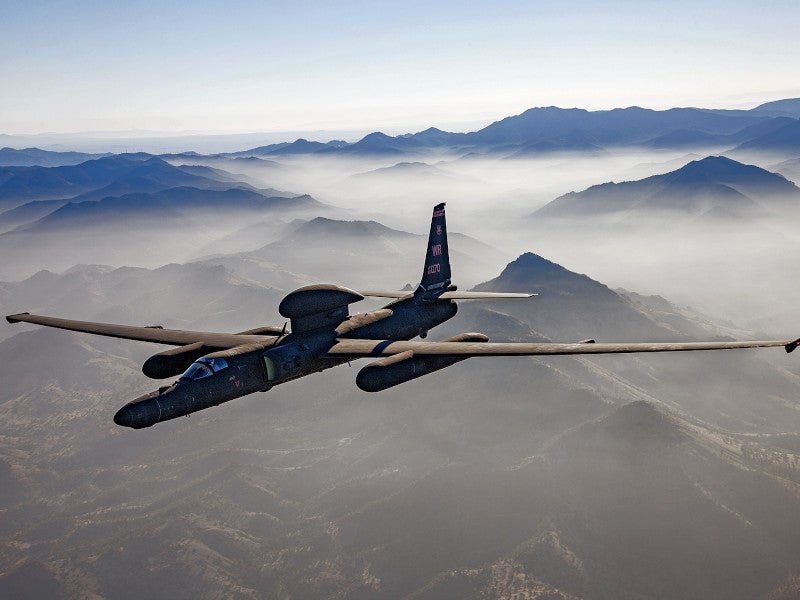The photograph showcases a small, dark military jet, possibly a vintage warplane, soaring over a dramatic mountainous landscape. The aircraft appears to have a sleek, elongated body with long, wide wings and several distinct tubes along its sides. The jet is primarily black and features a clear, slightly blue-tinted cockpit window at the front, through which the pilot can faintly be seen. On the tail of the jet, the letters "WR" are prominently visible, accompanied by the partial numbers "070" in pink. The plane is high in the sky above snow-capped peaks, with a sea of clouds and fog enveloping the lower parts of the mountains, adding a mystical layer to the scene. The mountains themselves are dark and textured, suggesting a rugged terrain, likely reminiscent of the Andes. Overall, the image captures the jet in flight, set against the vast, ethereal backdrop of sky and mountains.